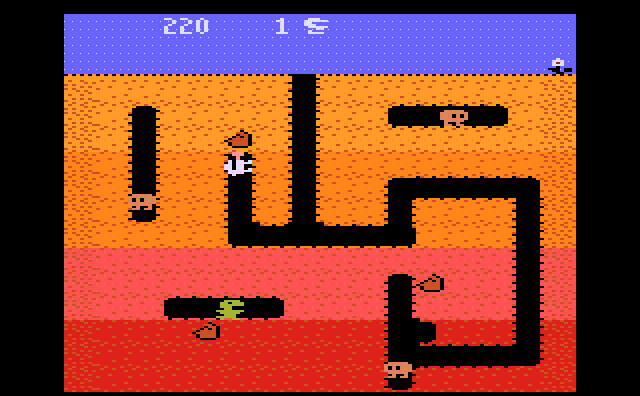This is an image of a video game centered around tunneling mechanics. The player starts at the top, where a blue section appears to be outside the main play area. From there, the game proceeds downwards through distinct horizontal layers of varying colors. These layers, in descending order, are light yellowish-orange, a deeper orange, a pinkish coral, and finally red at the bottom, possibly indicating increasing difficulty or danger as the player digs deeper. Within these strata, the player encounters various objects, some of which may present challenges or rewards, suggesting a strategic element to either avoid or collect them. The game interface shows multiple lives at the top of the screen, indicating that players have several chances to navigate through the layers. The precise objective of the game remains unclear, but it evidently involves a combination of exploration, strategy, and survival.